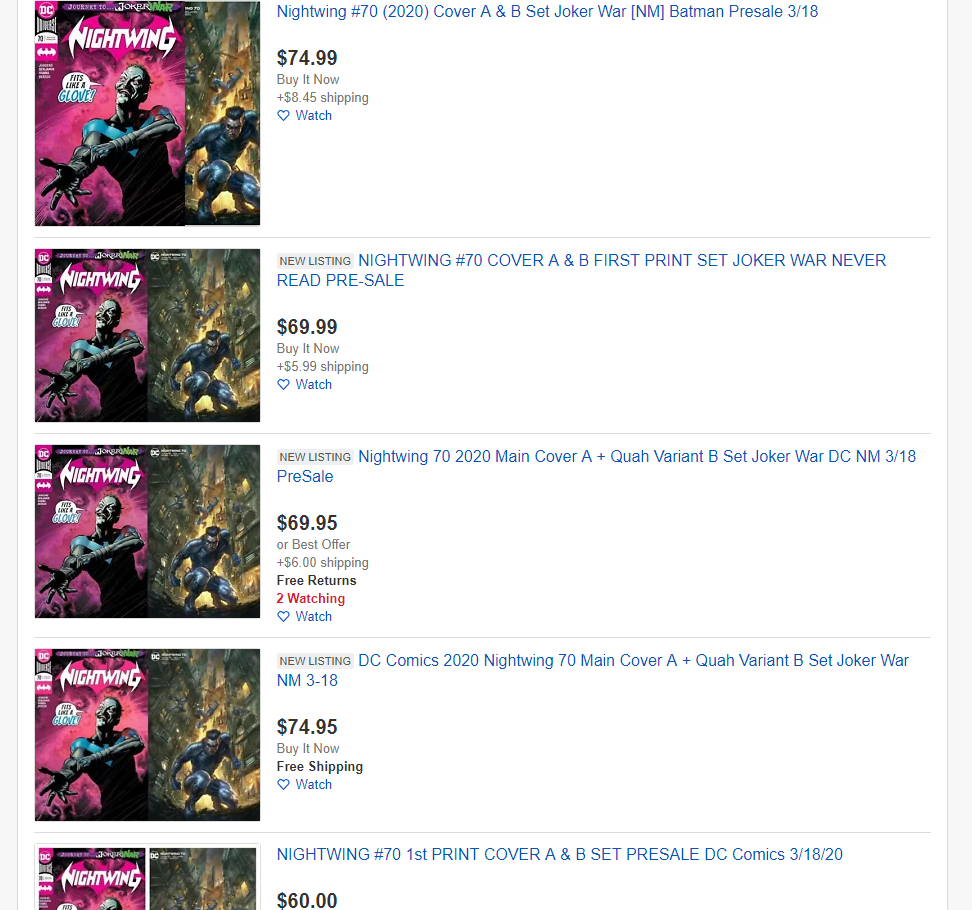This is a detailed screenshot of a web page from eBay featuring multiple listings for "Nightwing Issue #70" from DC Comics, specifically covering both Cover A and Cover B from the Joker War arc. There are five listings visible for the same comic book issue. The prices for these listings are as follows: $74.99, $69.99, $69.95, $74.95, and $60. Each listing is accompanied by identical images to the left. These images highlight the two variant covers for Nightwing Issue #70. 

The first cover, presumably Cover A, features the Joker standing against a pink background, dressed in Nightwing’s signature black and blue costume, with a speech bubble that reads, "It fits like a glove." The second cover, likely Cover B, portrays Nightwing crouched in what appears to be a scene from the gritty cityscape of Gotham. The juxtaposition of these covers accentuates the narrative tension in the Joker War arc, offering collectors two evocative pieces of artwork for this pivotal comic book issue.